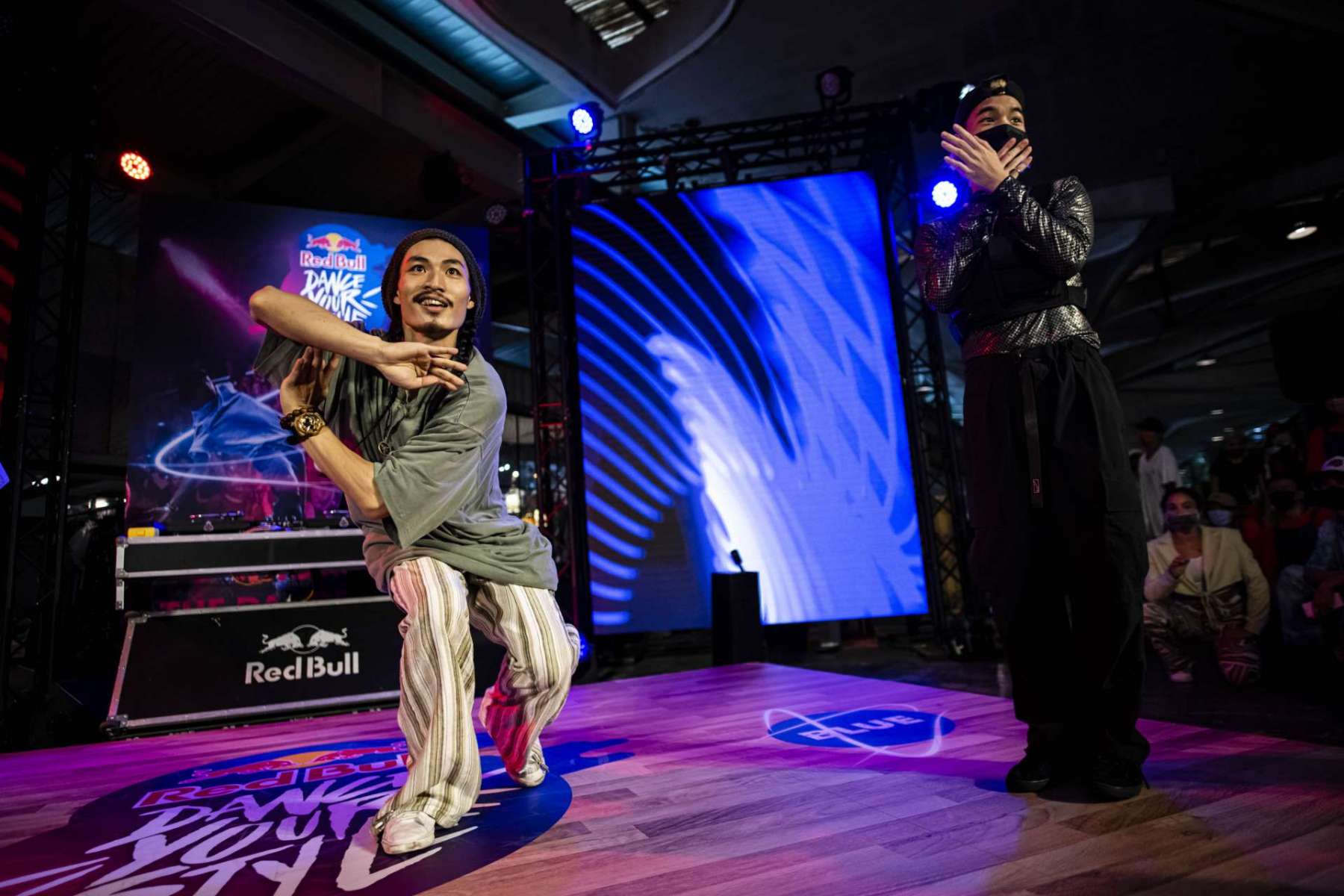In this vibrant image, two male performers are captured mid-dance on a wooden stage in what appears to be a club setting. The backdrop features a large, illuminated screen displaying "Red Bull Dance Tour," indicating the event is sponsored by Red Bull. Behind the performers, there is a DJ table prominently adorned with Red Bull logos. The dancer on the left is crouched down, sporting a gray t-shirt, brown and white striped pants, and white gym shoes, with what appears to be braids in his hair. The performer on the right stands with his arms crossed, wearing a black jacket, black pants, a reversed black baseball cap, and possibly a mask. The stage is buzzing with a purple-bluish hue from the vibrant lights, enhancing the lively atmosphere. You can spot a few audience members in the background, engrossed in the dynamic performance unfolding before them.